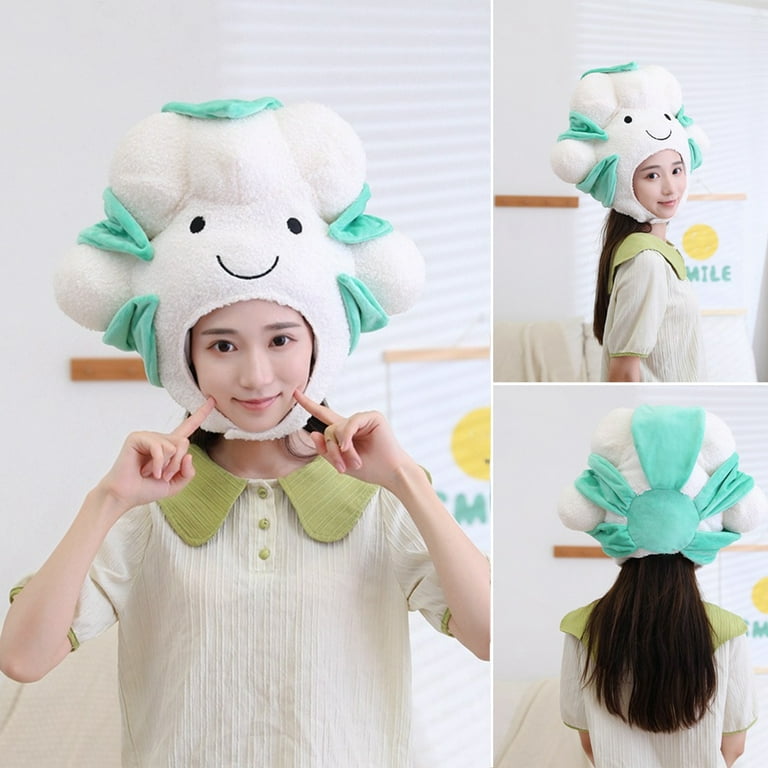The photograph is a high-quality image grid featuring a young Asian woman, likely Japanese and described as "kawaii" (cute in Japanese), modeling a unique hat. The overall grid includes three perspectives: one larger image on the left showing a frontal view, and two smaller images on the right depicting her from different angles. 

In the larger image, the woman is wearing a fluffy cloud-shaped hat with a smiley face, characterized by two black eyes and an open mouth. She touches her cheeks with her pointer fingers, creating dimples, and smiles brightly at the camera. The hat includes green accents, which wrap around the cloud shape and are visible in the other angles of the hat.

The top right image offers a side view, showing her facing to the right but still looking towards the camera, while the bottom right image provides a rear view, revealing a green sun on the back of the hat. The woman has long brown hair and is dressed in a textured white shirt with a green collar and buttons. The background is softly lit and entirely white, accentuating her playful and happy expression, along with the whimsical and cartoonish aesthetic of the cloud hat.